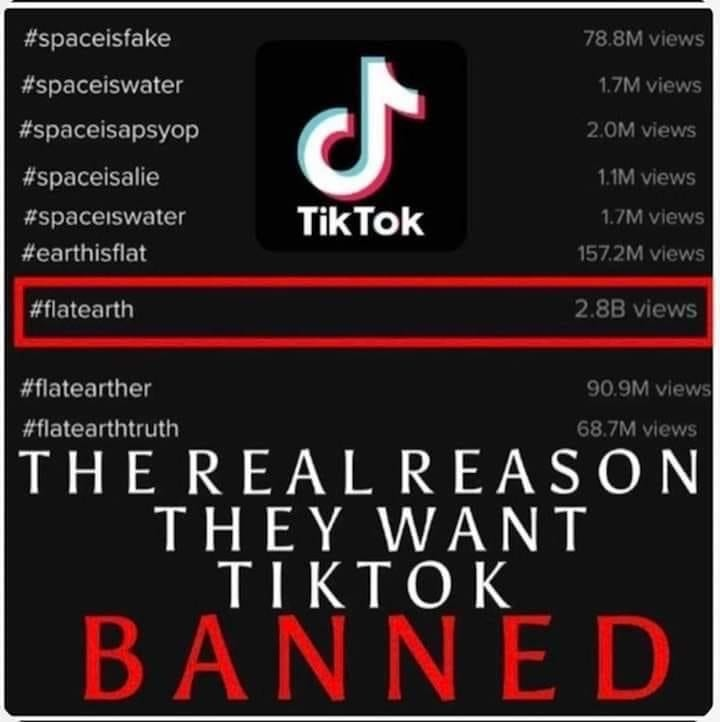Here is a cleaned and detailed caption for the image:

---

This image appears to be a screenshot of a TikTok video thumbnail with a completely black background. Positioned at the top center is the recognizable TikTok logo. 

The thumbnail prominently features a series of hashtags, each paired with view counts:
- On the left side: 
  - #spaceisfake (78.8 million views)
  - #spaceiswater (1.7 million views)
  - #spaceisapsyop (2 million views)
  - #spaceisalie (1.1 million views)
  - #earthisflat (57.2 million views)
  - #flatearth (2.8 billion views; this hashtag is outlined in a red rectangle)
  - #flatearther (90.9 million views)
  - #flatearthtruth (68.7 million views)

Beneath these hashtags, the text "the real reason they want TikTok" is prominently displayed in bold white uppercase letters. Below this phrase, the word "BANNED" is written in bold red capital letters. 

All the text on this thumbnail is in lowercase except for the final statement, which emphasizes the supposed reason for wanting TikTok banned. 

This thumbnail captures a provocative and conspiratorial theme focusing on controversial topics related to space and flat Earth theories.

---